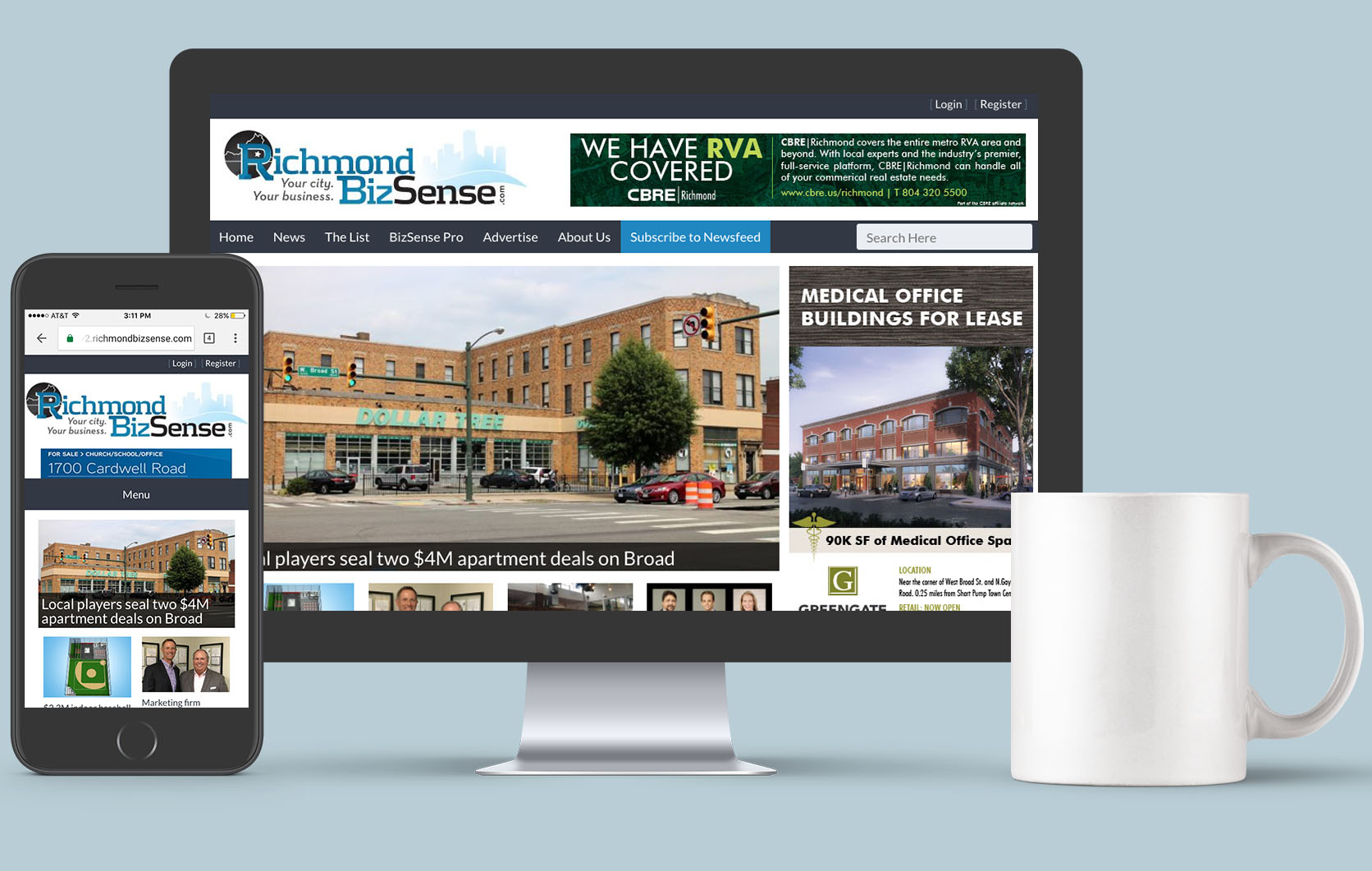In the image, a sleek modern workspace is meticulously arranged with a laptop, smartphone, and a plain white coffee cup positioned next to each other. The laptop and smartphone screens both display the Richmond Biz Sense website, which features the tagline "Your City, Your Business." Dominating the screen is an image of a large Dollar General building with cars parked in front of it. The website interface includes navigation options such as Home, News, The List, Biz Sense Pro, Advertise, About Us, and Subscribe to Newsfeed. Additionally, the laptop screen shows another image of a medical office building available for lease. The white coffee cup is situated to the right of the laptop, adding a touch of simplicity to the setup. At the top of the laptop display, the phrase "We Have RVA Covered" is visible, followed by clickable links and partially cut-off images. The scene suggests a productive environment, possibly enhanced by strategic use of Photoshop to create a polished, professional look.